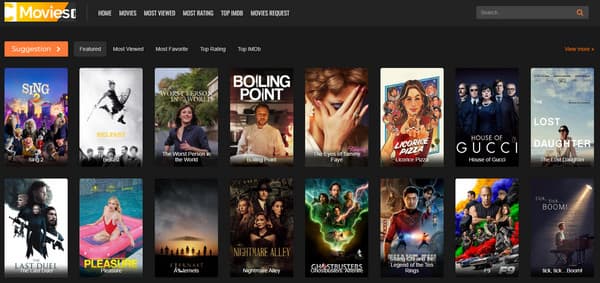A screenshot from the "Moviest" website is shown, with the site name prominently displayed at the top. Below the site name, there is a horizontal navigation bar with several options, including 'Home,' 'Movies,' 'Most Viewed,' 'Most Rating,' 'I-C-P-I-M-C-A,' and 'Movie Suggestions.' The navigation text appears blurry and pixelated, making it challenging to read, especially when the image is resized. An orange button labeled 'Suggestion' and a black button labeled 'Featured' are also visible in the top section of the site.

Immediately below the navigation bar, there are two rows of movie thumbnails, each containing eight movies. In the first row, the visible movie titles are "Sing," "I'm Not Certain," "Boiling Point," and "Licorné Pizza," with the remaining titles being too blurred to decipher. The second row includes titles such as "The Lost Daughter" and others that are partially indistinguishable due to the poor image quality.